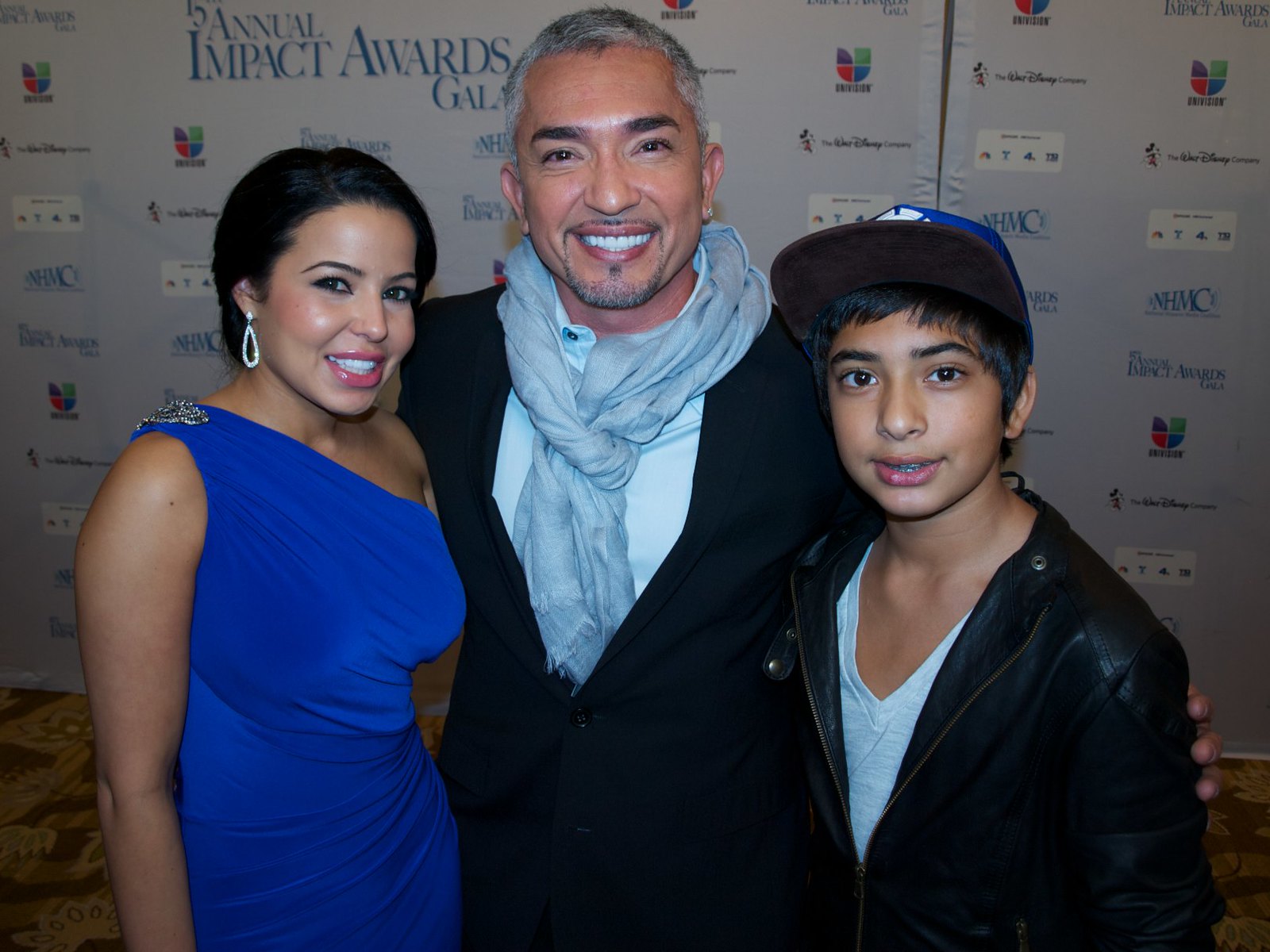This is a color photograph featuring three people posing together at the Annual Impact Awards Gala. On the left is a woman in a blue one-shoulder dress with a silver accent on the strap. She is smiling warmly at the camera, with her black hair elegantly tied up. Her accessories include teardrop-shaped diamond earrings. In the center stands a man with his arms around the two people beside him. He has short, gray-and-white hair, a neatly trimmed gray goatee, and is wearing an earring on his right ear. His attire consists of a black suit jacket, a light blue dress shirt, and a light blue scarf draped around his neck. On the right is a young boy with short black hair, dressed in a blue baseball cap, a light blue V-neck T-shirt, and a black leather jacket. The backdrop is a wall covered in various logos and text, including blue text on the upper left that reads "Annual Impact Awards Gala." All three individuals are smiling, creating a warm and unified scene.